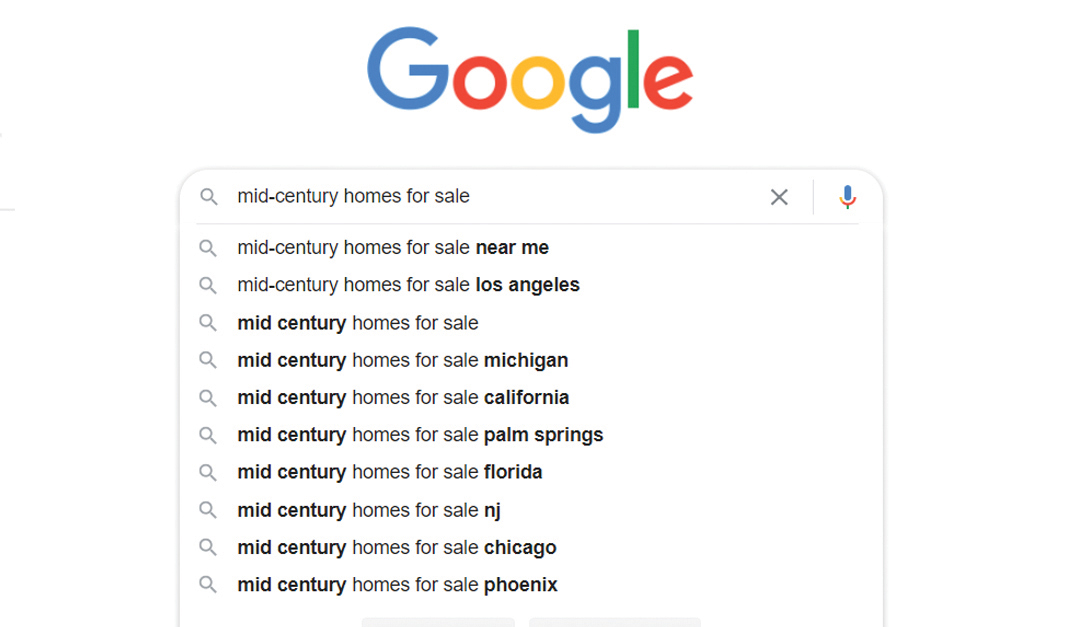This image showcases a screenshot of the Google homepage, dominated by the iconic "Google" logo in vibrant, multi-colored letters prominently displayed at the top center. Directly below the logo, there is the familiar search bar with rounded edges designed for inputting queries. On the left side of this search bar, there is a magnifying glass icon symbolizing the search function. Within the search bar, the text “mid-century homes for sale” has been typed. To the right of this input text, there is a small 'X' icon for clearing the search, followed by a microphone icon for voice search capabilities.

Below the search bar, a list of suggested search queries appears, each prefixed by a small magnifying glass icon. The top suggestion reads "mid-century homes for sale near me," followed by sequential location-specific variants such as "Los Angeles," "Michigan," "California," "Palm Springs," "Florida," "New Jersey," "Chicago," and "Phoenix." These suggestions provide users with relevant, related search options.

At the very bottom of the image, partially cut off, there appear to be two gray buttons which are likely the "Google Search" and "I'm Feeling Lucky" options, standard on the Google homepage but not fully visible in this particular screenshot. The overall image captures the quintessential search experience on Google, with a focus on mid-century homes for sale in various locations.